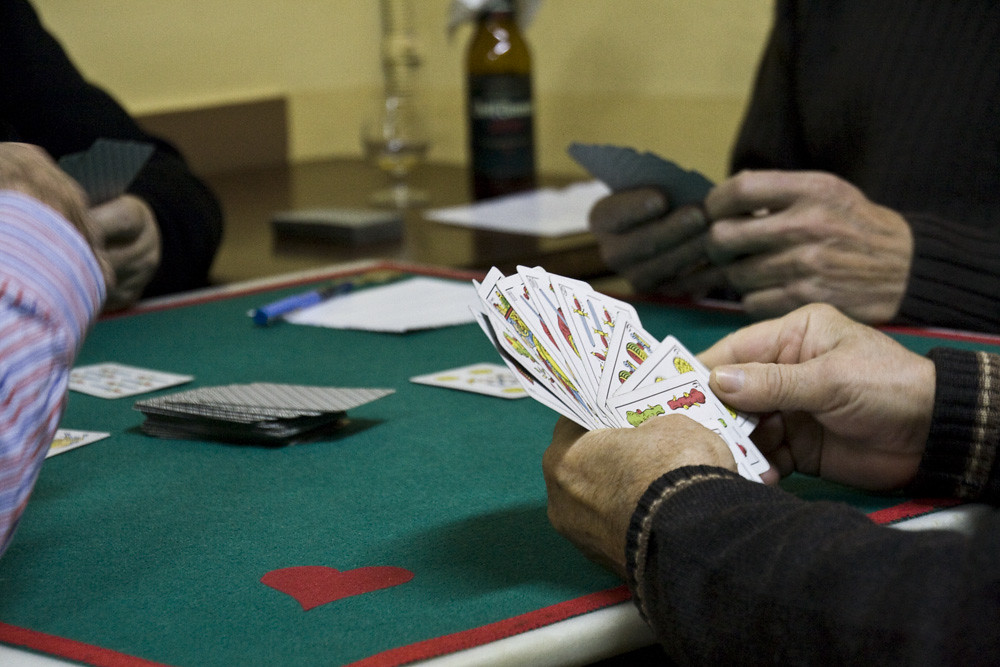A group of four elderly individuals are engrossed in a card game, seated around a square table with a green felt top, highlighted by red outlines and a red heart emblem in the center. Each player occupies one side of the table, holding a hand of cards. The scene is populated with various card game elements: a face-down stack of cards in the center and a scattering of face-up cards around the table. One player, situated in the bottom right corner, reveals their cards to the viewer. The participants are dressed in long-sleeved attire, comprising sweaters and a button-up shirt. A piece of paper and a pen lie in one corner of the table, suggesting scorekeeping or perhaps rules. In the background, another wooden table holds a wine bottle and a glass, next to which rests another sheet of paper and potentially another deck of cards. A lone chair is positioned at the rear of this secondary table, implying a readiness for more players or an upcoming game.